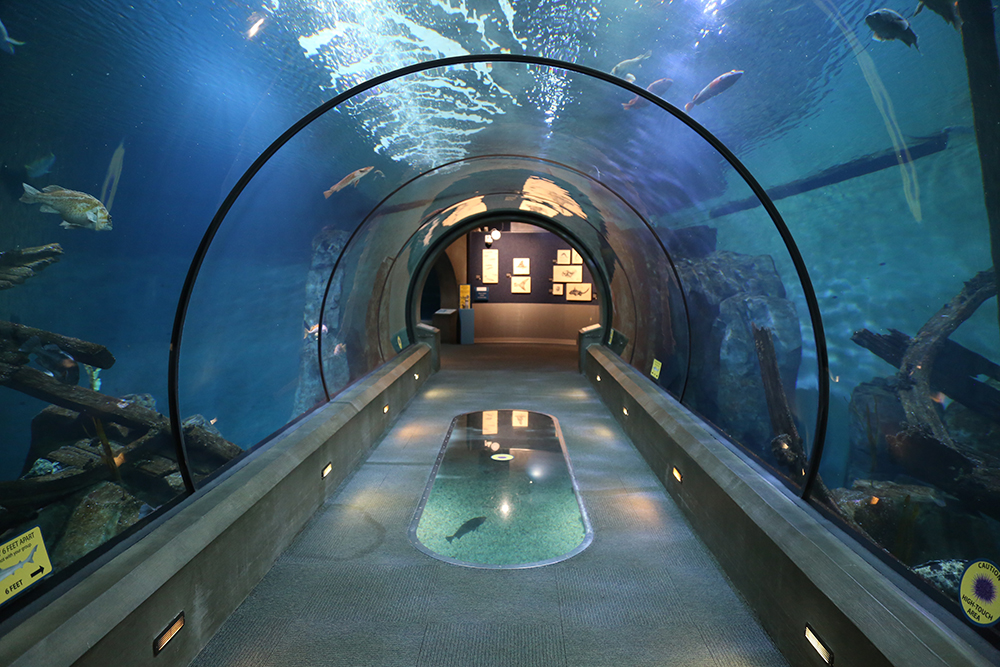This image showcases a mesmerizing underwater tunnel inside an aquarium, characterized by its large, arched glass windows that offer a panoramic view of the aquatic world surrounding it. The tunnel's walkway, which is gray and carpeted, is accentuated with small lights lining the edges and features a transparent floor panel that reveals fish swimming beneath, providing an immersive experience of an underwater seafloor, dotted with what appears to be debris and rocks, suggesting a shipwreck theme.

The tunnel is teeming with various species of fish, some identifiable like tiger fish with their distinctive orange and white stripes, and others that are either long and slender or robust like bass. The aquatic environment around the tunnel is brightly illuminated, especially at the peak, possibly due to strategically placed lighting or thinner water layers, enhancing the visibility of the vibrant marine life above.

At the far end of the tunnel, the passage opens into what appears to be another section of the aquarium. Here, a bulletin board illuminated with a yellow light displays artworks or information about different fish species. This area might also feature a seating area for visitors to rest and enjoy the view further. The entire tunnel structure, held together by strong black borders, invites visitors to marvel at the underwater spectacle both above and below, making it an enchanting pathway through the aquatic realm.